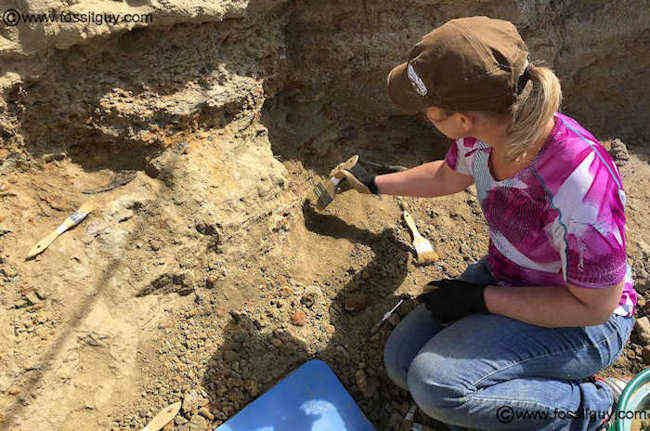In this detailed image, we observe a young woman deeply engaged in an archaeological excavation within a dry, desert-like site. The ground around her is entirely brown and sandy, devoid of any greenery. She is seated on the rugged terrain, her legs tucked in behind her as she focuses intently on brushing the dirt and stones. Dressed appropriately for her task, she wears blue jeans, a purple and white t-shirt, and black gloves. Her fair skin and blonde hair, secured in a ponytail, are partially concealed by a brown cap.

The woman's expression is not visible, as she is absorbed in her meticulous work, her eyes trained downward toward the ground. She holds a thick paint brush, actively sweeping dust and debris off the rocks in front of her. Surrounding her, a variety of tools and multiple brushes are scattered on the ground, indicative of her thorough preparation and methodical approach to the excavation. 

Among the scattered items, a blue tray lies on the ground just before her, its purpose uncertain. As she works, a tablet rests beside her, likely used for recording her findings and observations. The image further indicates its source, with a web link "www.fossilguy.com" discernable in both the upper left and bottom right corners, confirming its origin despite the slightly obscured text in the top left.